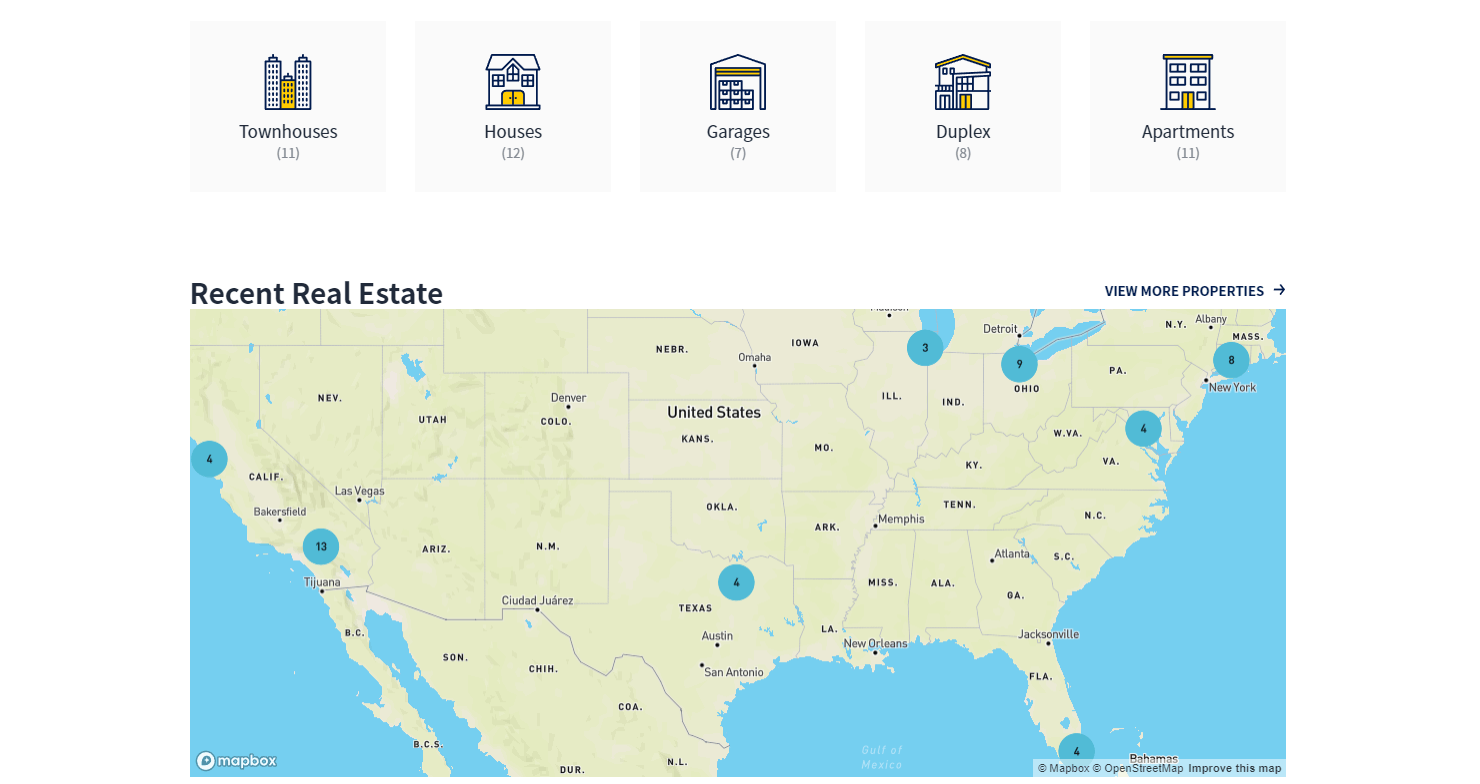A screenshot featuring a white background showcases various types of housing units and a real estate map of the United States. Within the image, there are 11 townhouses, each with 12 garages, and 7 duplexes. In addition, the image includes 8 apartments and 11 individual houses. The focal point is a detailed illustration of a townhouse complex, consisting of three connected buildings, with the middle one painted yellow. The houses are typical residential structures, while the garages are depicted as standard automotive storage units. The duplexes appear as single homes divided into different sections, and the apartments resemble typical multi-unit residential buildings.

Above the illustration, there is a map highlighting recent real estate listings across the United States. The map features an arrow to the right labeled "View More Properties." Various states are marked with numbers indicating the quantities of current listings: Florida has 4, Texas has 6, California (or possibly Virginia) has 13 and 4, New York has 8, Illinois has 3, and Ohio has 9. Some of the markings are difficult to read due to slight blurriness.